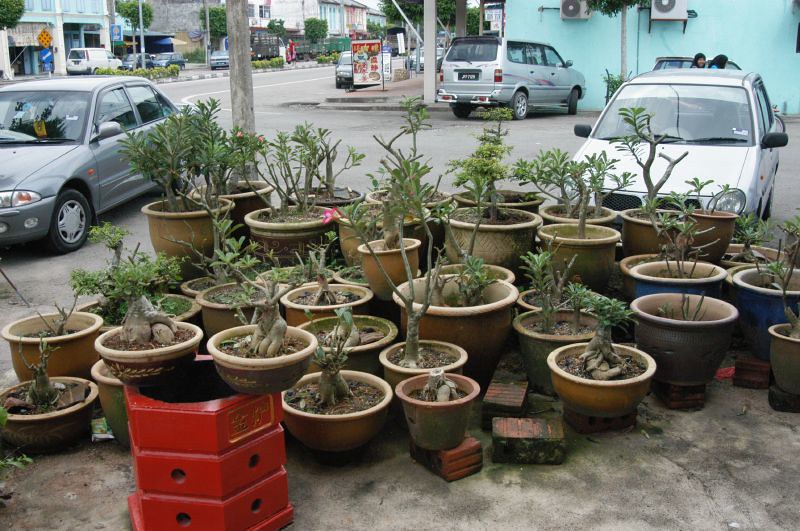This image captures a vibrant street-side display, likely a shop in an Asian country, featuring an array of around 30 potted bonsai trees. In the foreground, various plants are housed in pots that range from light brown to gray, and some pots are perched on bricks to elevate them from the concrete sidewalk. Notably, there is a prominent red, hexagonal stand with gold Chinese characters, upon which a couple of bonsai plants are displayed. The pots contain mostly cacti, characterized by multiple stems and greenery at the top but no visible flowers. 

In the background, a bustling cityscape can be seen. Two cars are parked close to the display, one facing towards and the other facing away from the viewer. On the left side of the image, a person appears to be walking, while in the top right corner, two women with long dark hair are seen laughing and pushing a bike behind one of the parked cars. Additionally, there is signage in the background, likely indicating the presence of a restaurant, with characters that appear to be Chinese. The surrounding buildings are a mix of white, light blue, and light pink, and further in the distance, yellow and blue umbrellas can be spotted over café tables, indicating a lively urban environment.